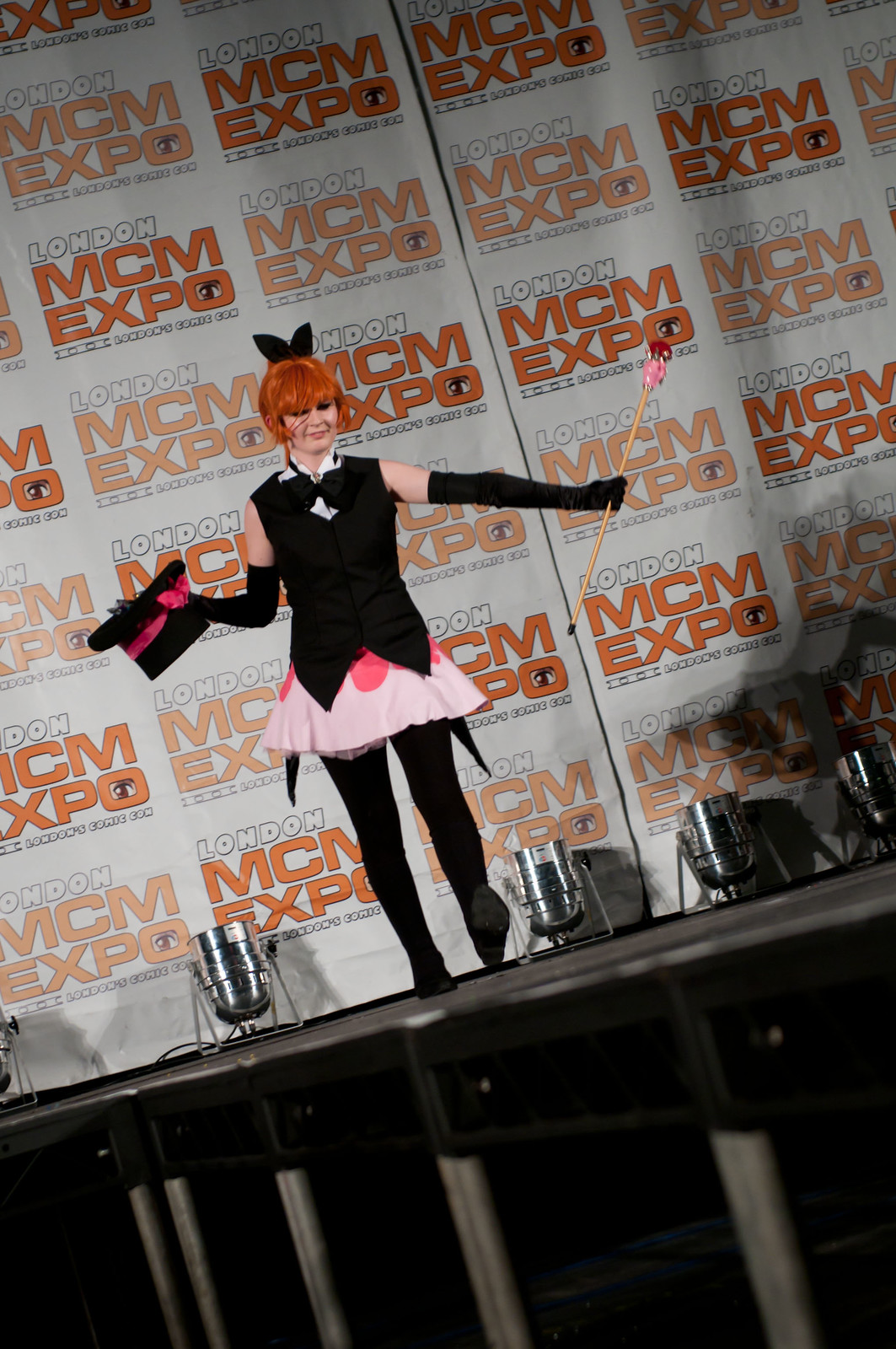The image features a woman standing on a black stage, clearly dressed in an elaborate costume reminiscent of a magician's assistant, a magician, or a bunny. She has vibrant, almost orange hair and is adorned with black bunny ears. Her outfit consists of a black shirt with a white collar and what seems to be a black bowtie, long black gloves that extend past her elbows, black tights, black shoes, and a pink skirt that layers over a darker pink, petal-like skirt. In her left hand, she holds a wand or baton with a pink tip, while her right hand grasps a black top hat featuring a pink stripe or bow. The backdrop behind her is a wall plastered with the text "London MCM Expo" repeated symmetrically multiple times, akin to a step-and-repeat banner found at red carpet events. The background has bright white lighting and is flanked by colander or tub-like objects on the ground. The camera angle is slightly tilted to the right, adding a dynamic perspective to the overall scene.